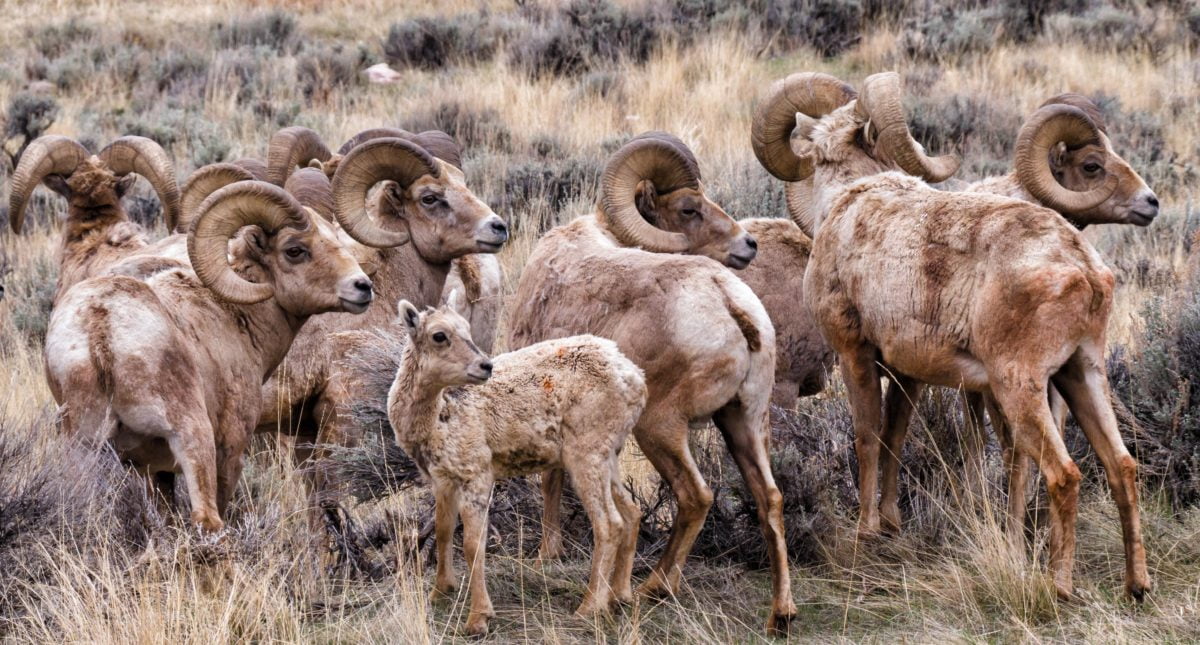The photograph captures a herd of bighorn sheep, comprising approximately eight or nine adults and one young lamb without developed horns, all standing in a dry, beige meadow during what appears to be a cloudy day. The adult sheep are distinguished by their tan-brown coloration and characteristic C-shaped horns. Both males and females are present, and they are arranged such that many are facing to the right, seemingly alerted by a common sight or sound. A young lamb in the foreground gazes in almost the same direction, adding to the sense of collective attention. The meadow is dotted with tall, dry grasses and low shrubs, possibly sagebush, with no green grass visible, signifying a likely arid environment. In the background, a white object with brownish-gold textures, resembling either a skull or a rock, further adds to the rugged, natural setting. This professional-quality image, likely taken by a wildlife photographer, encapsulates a peaceful yet watchful moment in the lives of these majestic animals.